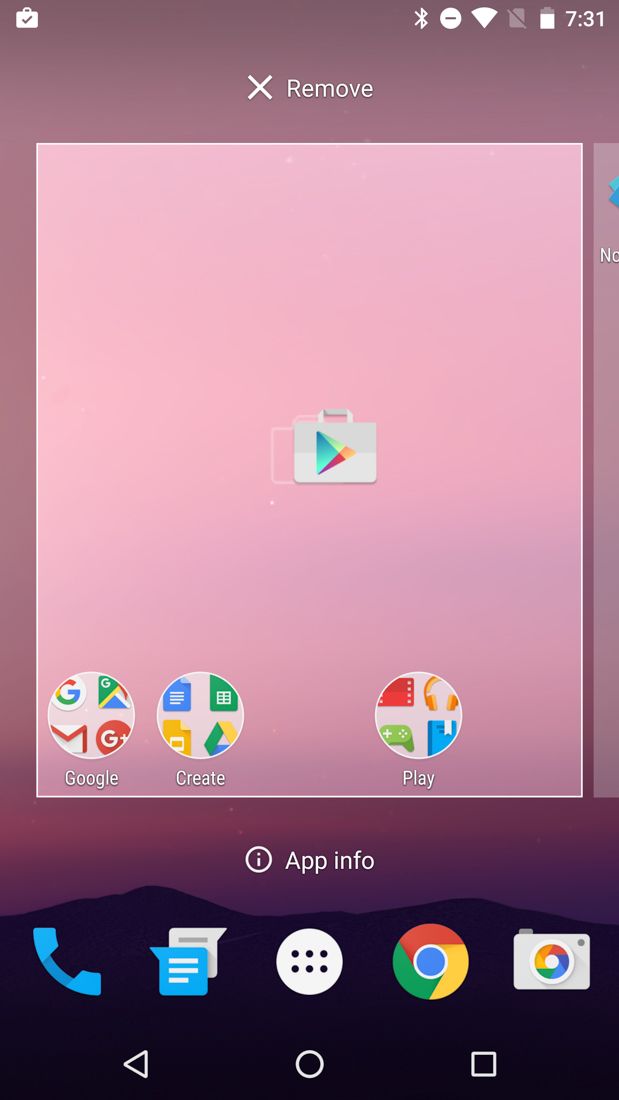The image depicts a cell phone screenshot featuring a gradient background that transitions from mauve at the top to a darker shade at the bottom. The darkened lower section resembles a mountain range, atop which five icons are positioned. These icons include (from left to right): a phone, text messaging, a home button, Google Chrome, and the camera.

In the upper left-hand corner of the screen, a white square with a check mark is visible. The top-right corner displays standard cell phone indicators such as signal strength, battery life, and the time. Approximately four lines below this, centered, is a white 'X' icon, accompanied by the word "REMOVE" in gray lettering.

Two lines below the 'X' is a large, square area outlined in white with a pale pink background, featuring the Google Play Store suitcase icon at its center. At the bottom of this section are additional icons: a Google icon, a 'Create' icon, a blank space for an icon, and a 'Play' icon.

Further down, approximately three lines below, a white circle outlined in white with a lowercase 'i' in its center appears. Adjacent to this icon, the text "APP INFO" is noted.